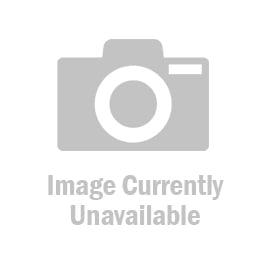This detailed image displays a close-up of an ENSTAT 2020 ionizing air blower. The entire background is stark white, emphasizing the white, rectangular mechanical structure at the center. This device is mounted on a white stand with black screws on both sides that allow it to pivot. The blower's front, oriented to the left, features a prominent fan situated within the top half. The fan is green and encased in a black metal or plastic frame that forms an X over it. Below the fan, text on the left side reads "Simcoe Ion," with 'Ion' enclosed in a blue circle. Adjacent to this text, within a blue rectangular section, is white text stating "ENSTAT 2020 IONIZING AIR BLOWER." This section also hosts two switches: a red power button labeled "Power" above it, and a black switch for adjusting fan speed, labeled "Fan Speed" above it. A black knob on the right side of the blower allows for manual adjustments.